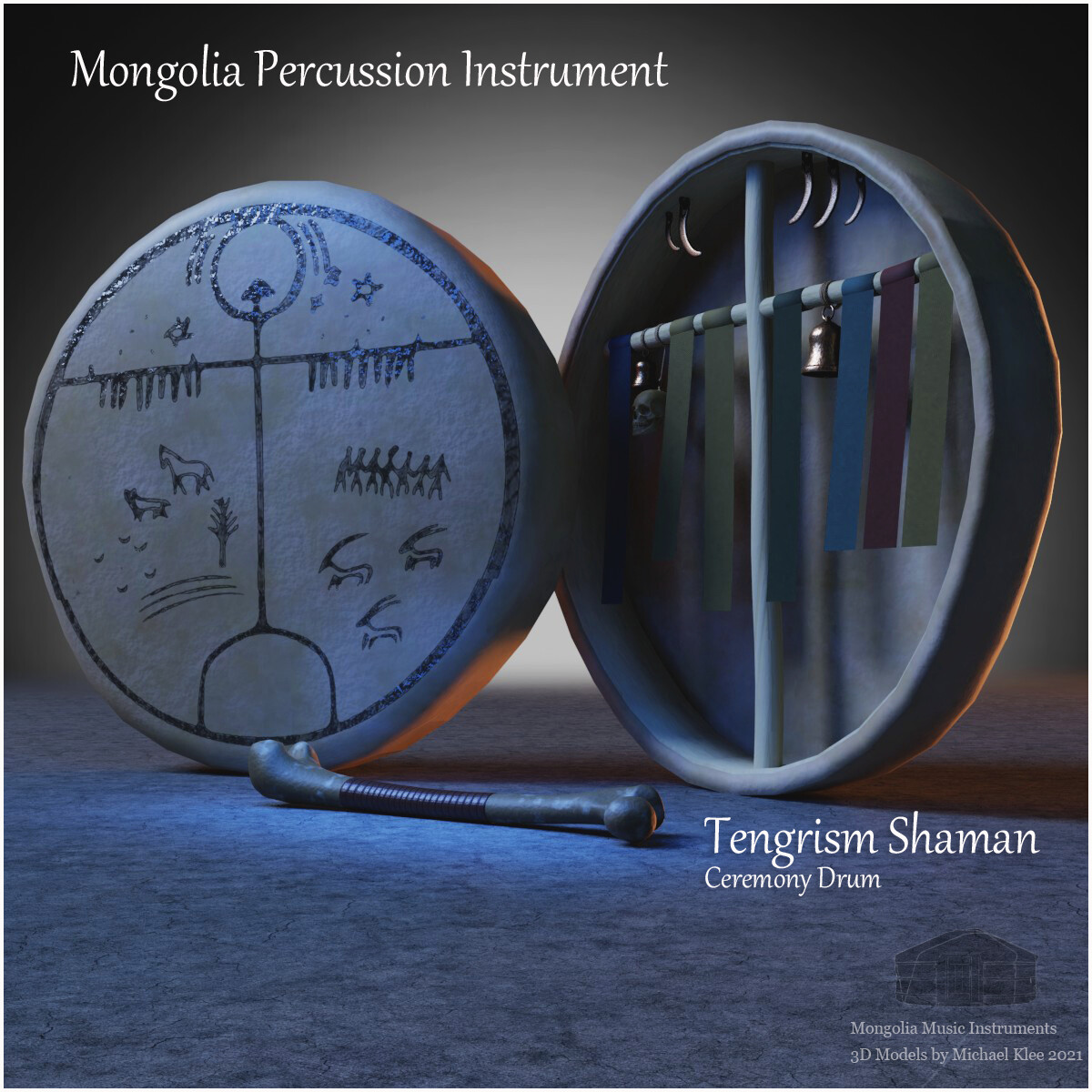The image showcases a highly detailed 3D model of a Tengrism Shaman Ceremony Drum, part of the "Mongolian Music Instruments" series created by Michael Klee in 2021. The drum, which is circular and features a rawhide front, is prominently displayed with intricate hand-painted imagery in black and white, depicting animals and traditional First Nations scenes and symbols. The top left of the image includes a label in white text reading "Mongolia Percussion Instrument," and the bottom right bears the description "Tengrism Shaman Ceremony Drum," while further down, in smaller text, it states "Mongolian Music Instruments 3D Models by Michael Klee 2021." The drum's interior reveals a wooden cross structure, adorned with bells, ribbons, and a metal rod, potentially used as a drumstick. The background of the image is suffused with dark, blue hues, giving the model a mystical, ethereal appearance.